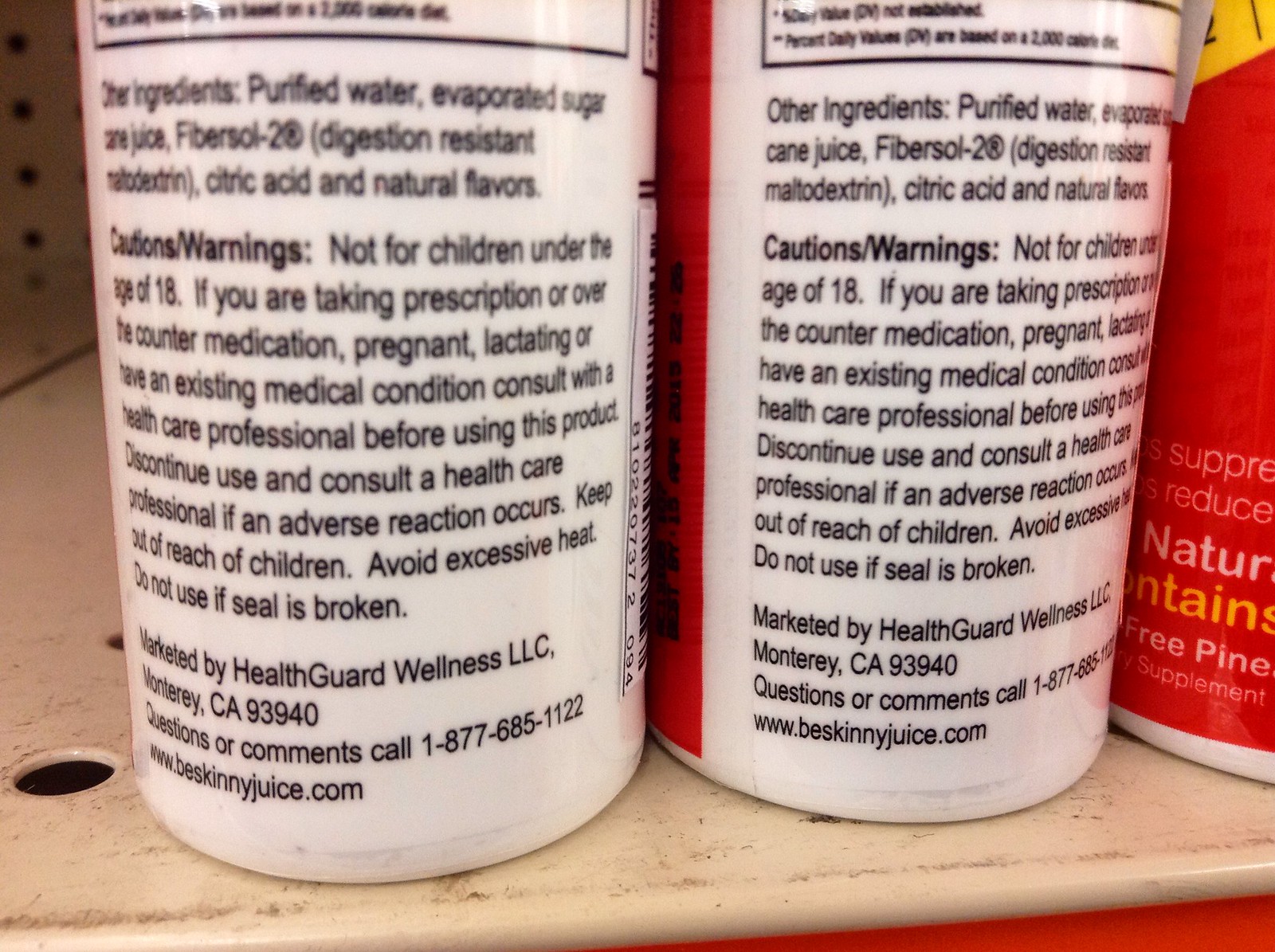This image showcases the back labels of two bottles, providing a detailed glimpse into their contents and manufacturing information. The black and white labels predominantly feature the list of ingredients, which include purified water, evaporated sugar cane juice, Fibersol-2, citric acid, and other constituents. The top portion of the label is cut off, but the remaining text indicates the bottles contain a beverage. The labels also reveal that the product is marketed by Health Card Wellness, LLC, based in Monterey, California. Additionally, contact information, including a phone number and a website, is displayed at the bottom of the labels. Both containers are identical in design and information.